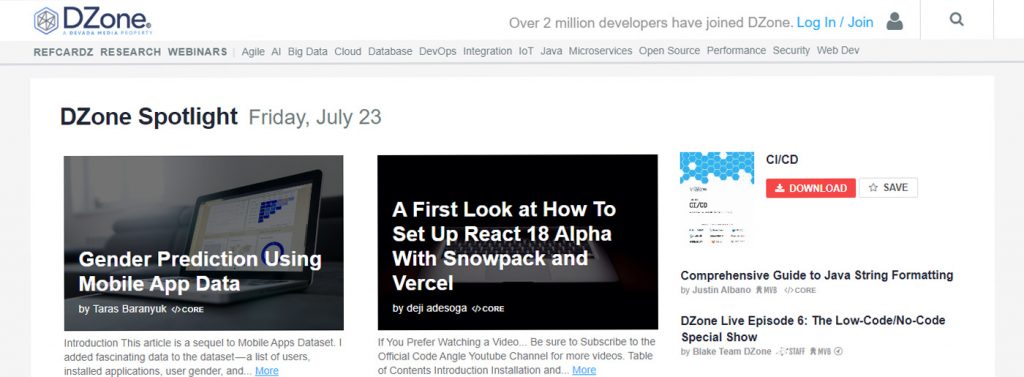The image is a screenshot taken from the top section of the D-Zone website, as indicated by the logo in the top left corner. The featured page seems to be dedicated to research webinars. In the top right-hand corner, there are options to log in or join the site, along with a search icon symbolized by a magnifying glass.

The main body of the webpage showcases a title that reads “D-Zone Spotlight, February, July 23rd.” Below this title are two clickable sections: one labeled "Gender Prediction Using Mobile App Data," and another titled "A First Look at How to Set Up React 18 Alpha with Snowpack and Vercel." To the right, there are additional articles available for exploration.

The website's background is predominantly white, providing a clean and simple aesthetic, while the text is rendered in dark black for clear readability. The overall design and content strongly suggest that D-Zone is a platform focused on presenting and facilitating research webinars and related materials.